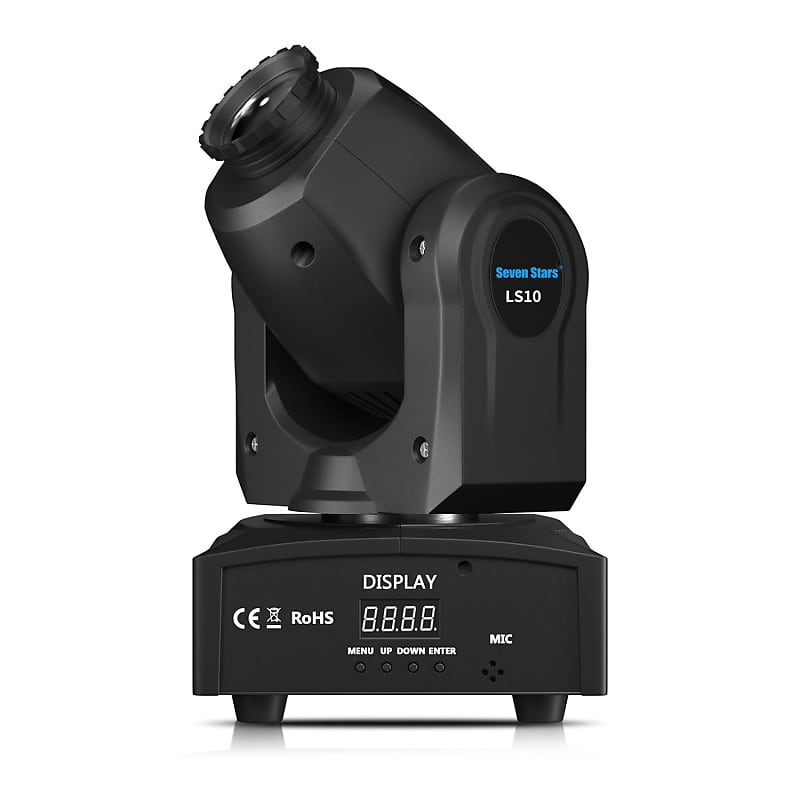The image depicts a Seven Stars LS-10 laser projector, featuring a sleek black design. The device has a rotatable top section that can be tilted to various directions, with a black lens encased at the apex. The projector is connected to a base with two small legs standing on a white surface. Clearly displayed on the side, the brand "Seven Stars" is written in blue, with the model number "LS-10" in white underneath. The base includes a detailed control panel featuring a digital display that shows '8888' when off. Below the display are four clearly labeled buttons—Menu, Up, Down, and Enter—along with a microphone port marked "Mic" surrounded by four small holes. Silver screws attach the various components, and the base prominently displays certifications "CE" and "ROHS."